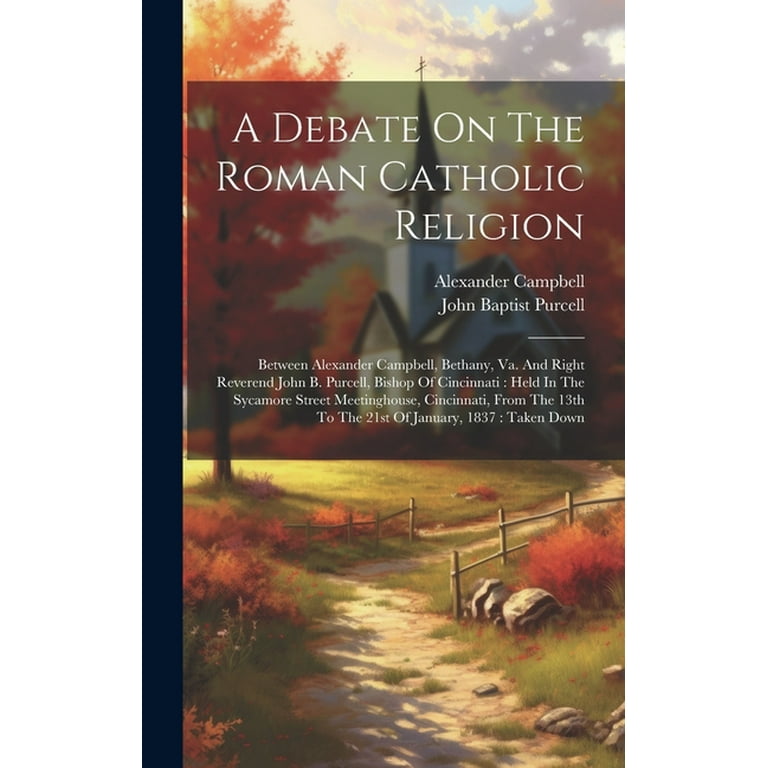The image is a color illustration of a book cover titled "A Debate on the Roman Catholic Religion." The cover features a picturesque countryside scene centered around a white church with a brown bell tower and a tall steeple topped with a cross. The church, framed by orange autumn trees, stands at the end of a winding dirt path bordered by wooden fences and rocks, adding to the rustic charm. Red bushes adorn the lower right corner, and the sky is a mix of gray and white hues.

A dark vertical stripe runs along the left binding side of the book, contrasting with the rest of the cover. The upper part of the cover features a semi-transparent black rectangle with white capitalized text detailing the book's title, "A Debate on the Roman Catholic Religion," and the authors' names, Alexander Campbell and John Baptist Purcell. Additional details, including the debate's location and dates, are also present, highlighting the historical 1837 debate held at the Sycamore Street Meeting House in Cincinnati.